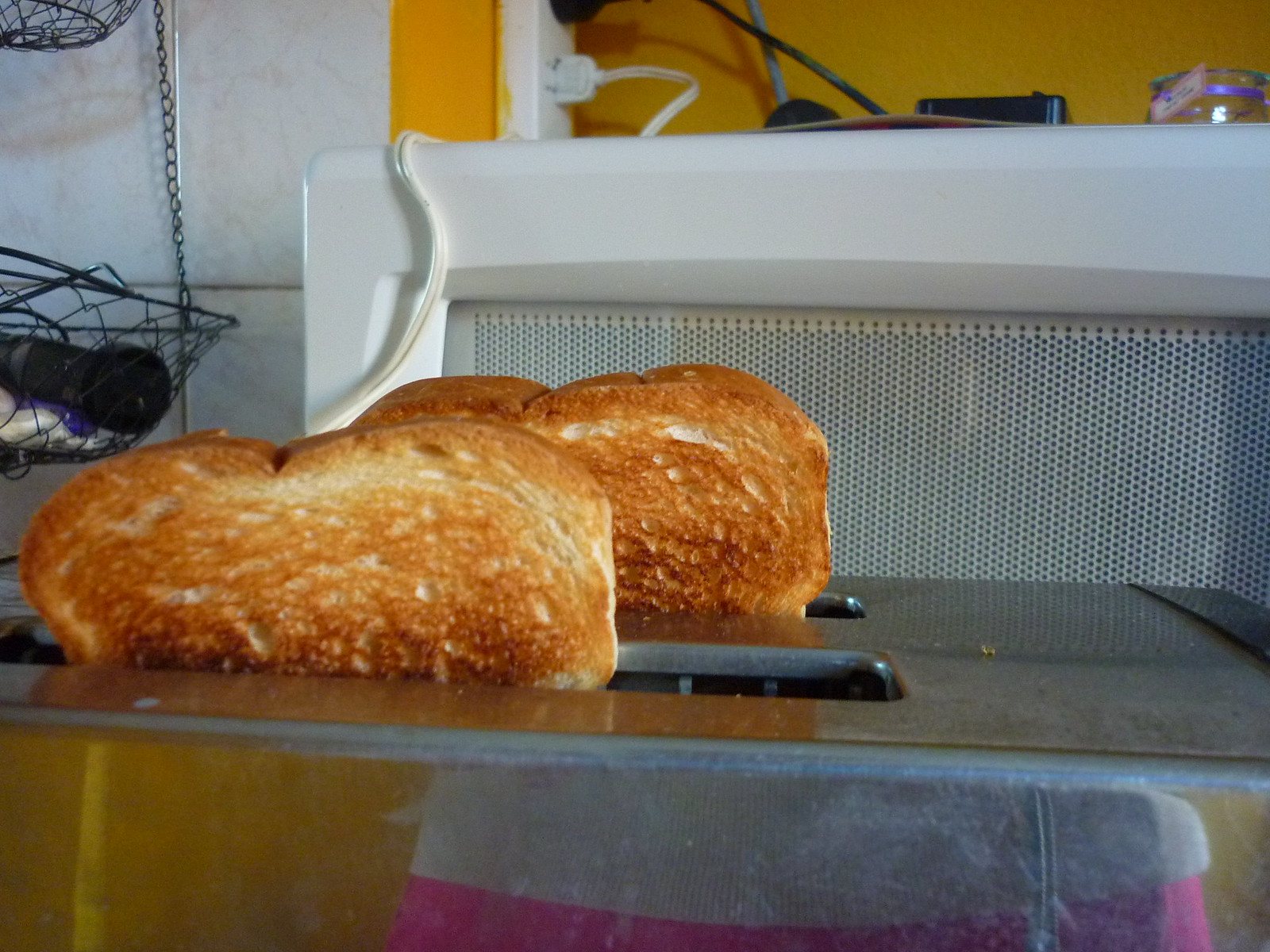This close-up image captures two golden-brown pieces of toasted white bread emerging from a stainless steel toaster, reflecting a pink and white object on its polished surface. The toaster's slots are clearly visible, with the crusts of the toast slightly darker. Positioned in a kitchen setting, the background features a white microwave with a screen and a yellow wall. Adjacent to this, a multi-level black wire basket is partially visible on the left, its lower basket containing black, white, and purple items. In the upper right corner, there's a jar adorned with a purple ribbon and tag. A white electrical outlet is seen with both a white and black cord plugged in.